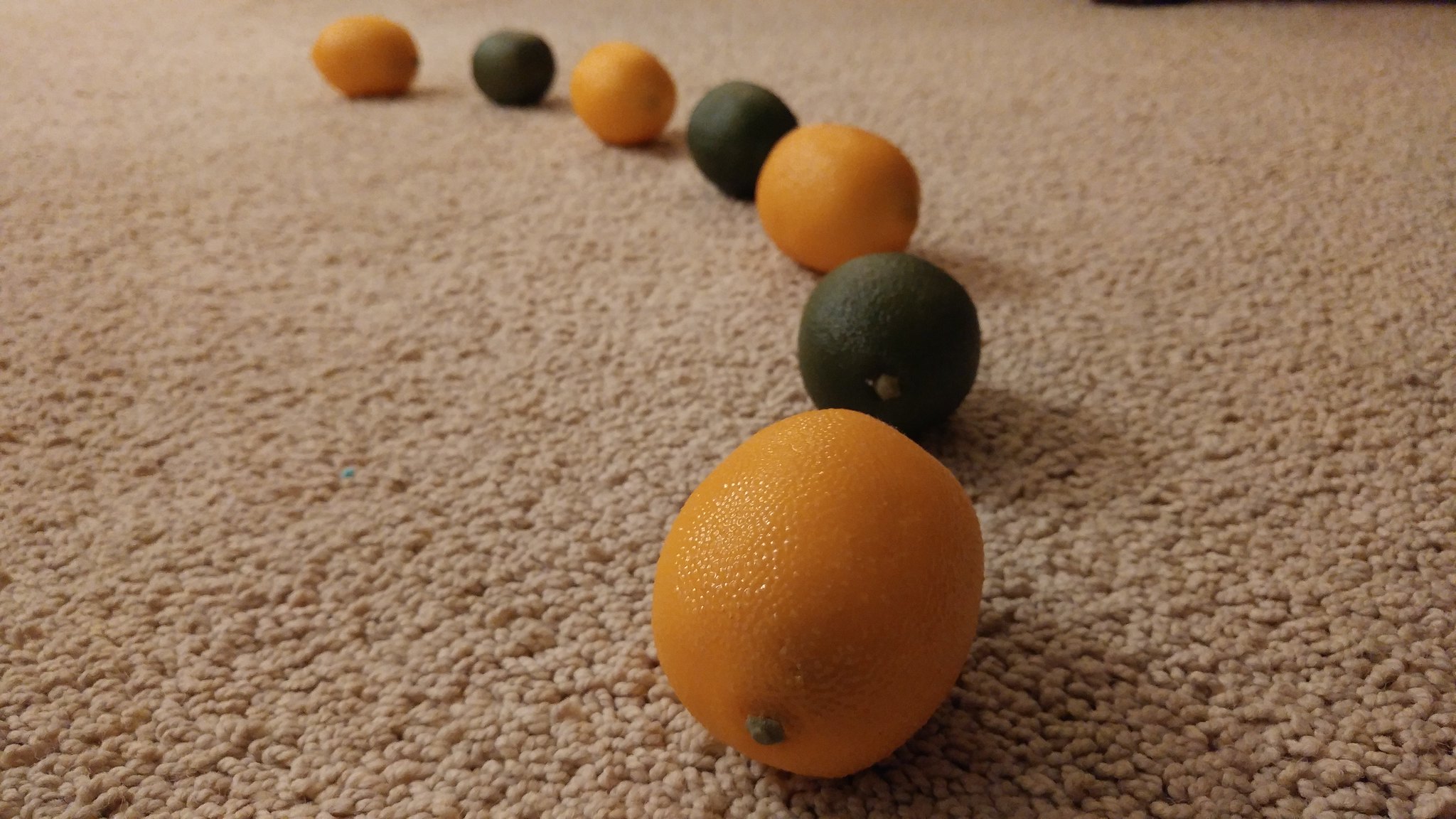The picture features a series of seven well-organized fruits, arranged in a curved line approximately a meter long, with small gaps between each. The fruits alternate between four oranges and three green limes, creating a visually pleasing pattern. Each fruit's stem is visible, and their shadows fall to the right, enhancing the composition. They are placed on a beige carpet, giving the scene a soft, inviting background. The wide-angle view captures the fruits arranged almost in a half-circle on the carpeted surface, showcasing the meticulous placement and vibrant colors.